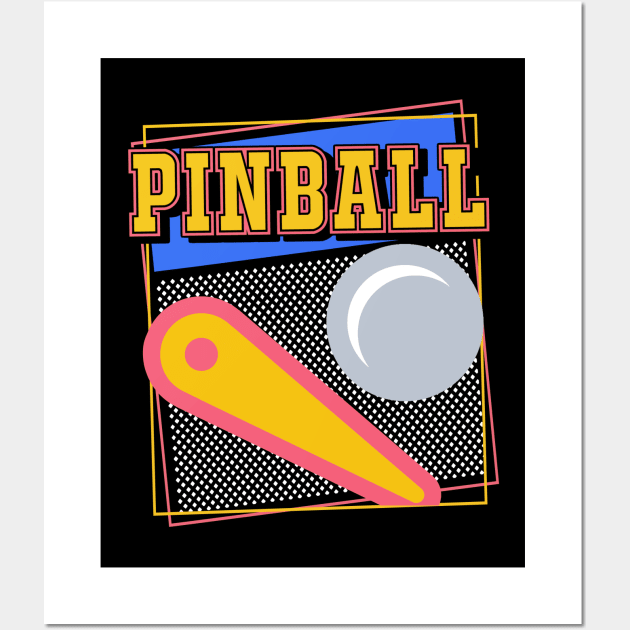The image depicts a retro-style poster against a gray background with a prominent white border. The poster itself features a black background and is almost square but slightly taller than it is wide. The focal point is the vibrant yellow text, outlined in pink and black, spelling out "PINBALL" at the top, superimposed on a slightly diagonal blue rectangle. Below the blue rectangle, the background transitions to a black and white polka dot pattern.

Adding to the retro aesthetic, the design within the black background includes overlapping rectangular outlines: an orange-yellow one and a skewed pink one. Central to the composition is a large, shiny gray pinball, positioned just beneath the word "PINBALL." Adjacent to this is a stylized pinball flipper, colored yellow on the inside and outlined in pink, situated lower and to the left of the pinball. The overall design is characterized by its bright neon colors set against the dark backdrop, invoking a nostalgic feel reminiscent of the classic pinball era.